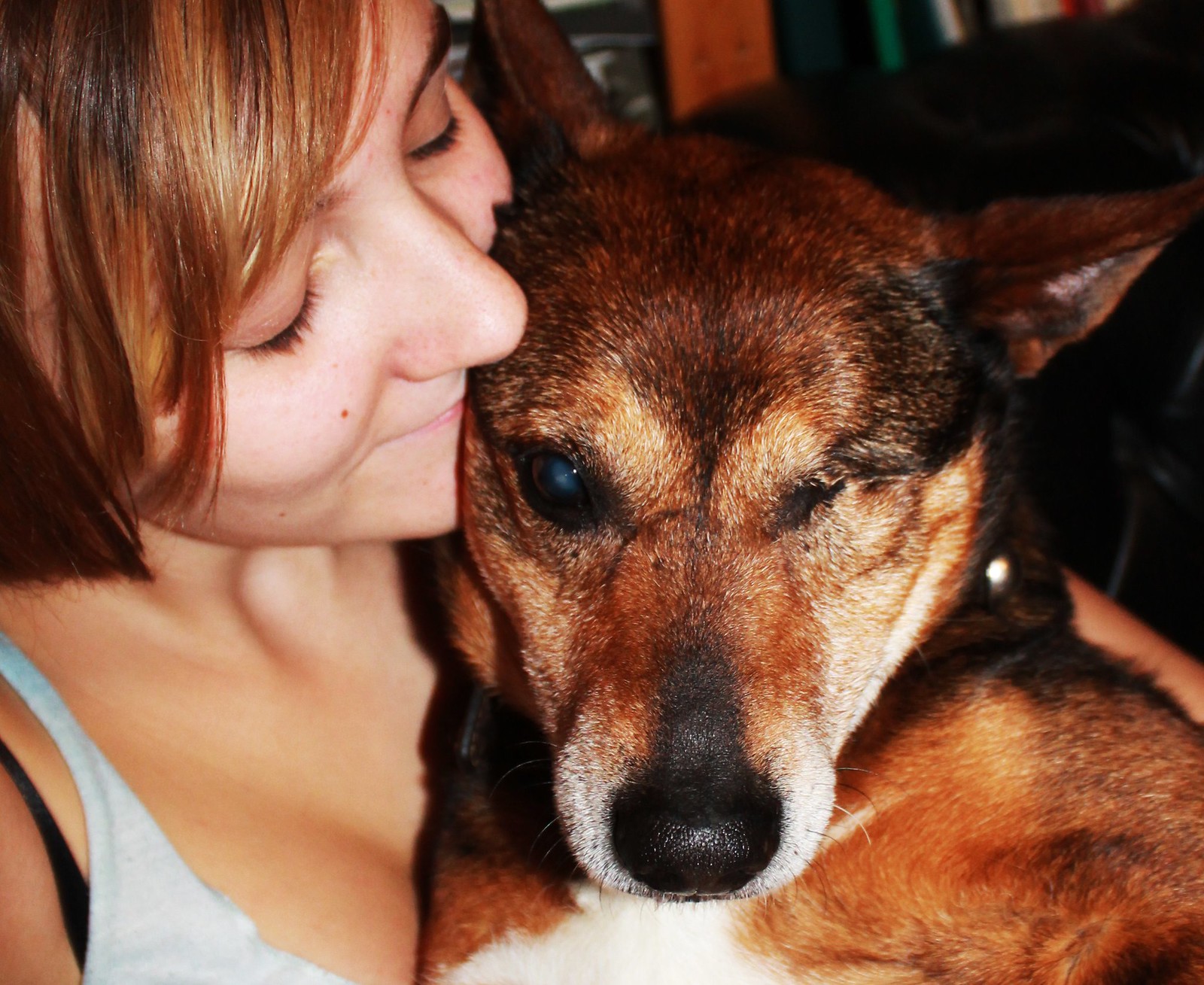In this close-up image, a woman with brown, highlighted hair and wearing a white tank top with a black bra underneath, lovingly holds a reddish-brown dog with short hair and pointy ears. The dog, which has a shiny black nose and white fur around it, appears to be missing its left eye and possibly has a cataract in its right one. The woman has her eyes closed and her cheek nuzzled against the dog's head, with her lips almost touching its forehead as if about to kiss it. The scene captures a tender moment, despite the dog looking a bit uncomfortable with the close snuggle.